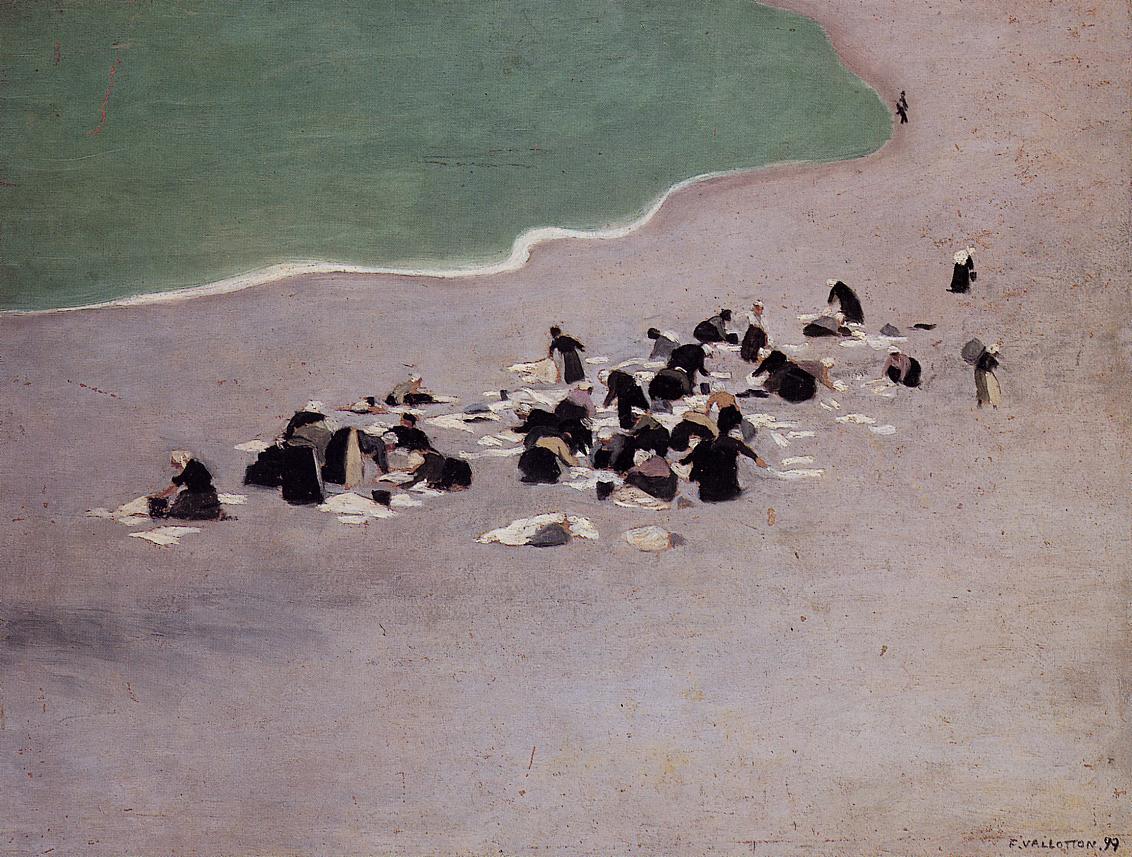This painting, titled "Washerwomen at Etretat" by Felix Valloton, captures a vivid coastal scene in a landscape orientation, utilizing a combination of realism and abstract art. The foreground is dominated by beige-pink sandy beach stretching from the top right to the bottom left of the frame. A group of women, dressed in black garments and aprons with their hair wrapped, are depicted laboring intensely. They are engaged in washing and drying white garments laid out across the sand, giving an impression of hardworking washerwomen, some of them seen kneeling over the fabrics, while others carry bundles on their backs. In the background, the pale green-blue ocean with scattered white foam can be seen gently lapping at the shore. The scene is set with various muted and neutral colors including black, white, gray, tan, brown, with hints of blue and green. The composition also includes minimalistic details, such as what appears to be a tiny signature in the far bottom right corner. The painting skillfully portrays the diligence and communal efforts of these women against the scenic coastal backdrop.